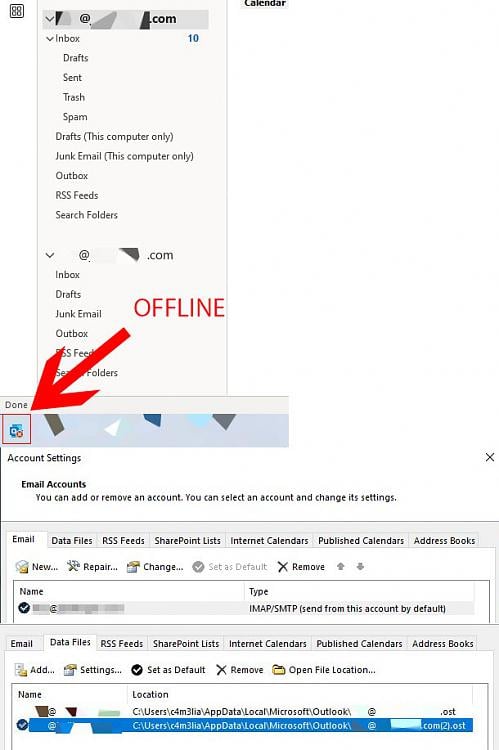**Detailed Caption:**

The image is a screenshot of an email client interface, showcasing a side menu that appears to be part of a larger, web-based email management system. The central focus is on a pop-up window that has emerged from the main interface. A prominent red arrow points from the upper left-hand icon of the website to this side menu, suggesting a connection or action linked to this area. The pop-up side menu includes a list of email folders: Inbox, Draft, Sent, Trash, Spam, Drafts (This Computer Only), Junk Email (This Computer Only), Outbox, RSS Feeds, and Search Folders. 

At the top of the main screenshot, the word "OFFLINE" is displayed in bold, red capital letters, followed by the red arrow pointing to an indeterminate icon in the upper left corner. Below this, there are options for "Account Settings," "Email Accounts," and functionality to add or remove accounts, select accounts, and change settings. 

Tabs at the top of the window include categories such as Email, Data Files, RSS Feeds, SharePoint Lists, Internet Calendars, Published Calendars, and Address Book. Under these tabs, a blurred-out name is visible alongside the label "Type," which specifies "IMAP/SMTP (Send From This Account By Default)." 

Toward the bottom, there appears to be a duplicated set of the tabs mentioned earlier, and associated with these tabs are fields for a name and location, although specific details are obscured or blurred.